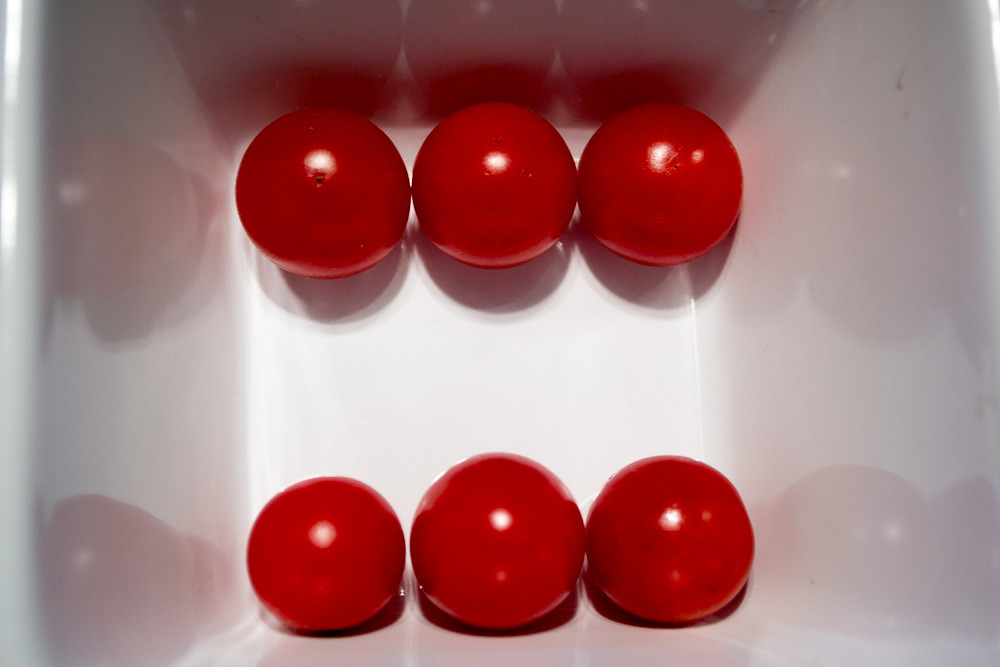The color photograph captures a top-down view of a deep, square-shaped, pale white or possibly silver bowl, bathed in light that reflects off its surfaces. Inside the bowl, two perfectly aligned rows of three bright red cherry tomatoes or grape tomatoes are neatly arranged. Each tomato in the top row touches its neighbors and is positioned close to the upper edge of the bowl, while the bottom row mirrors this arrangement along the bottom edge. The tomatoes are small, likely about an inch and a half to two inches wide, and exhibit flawless, smooth surfaces with a distinct, centralized flash of light. The bowl’s reflective surface enhances the visual appeal by casting subtle reflections of the tomatoes and the light onto its sides, adding depth and dimension to the photograph. Towards the bottom of the image, between the first two tomatoes, there appear to be two small metallic reflections or objects, adding a hint of mystery to the composition.